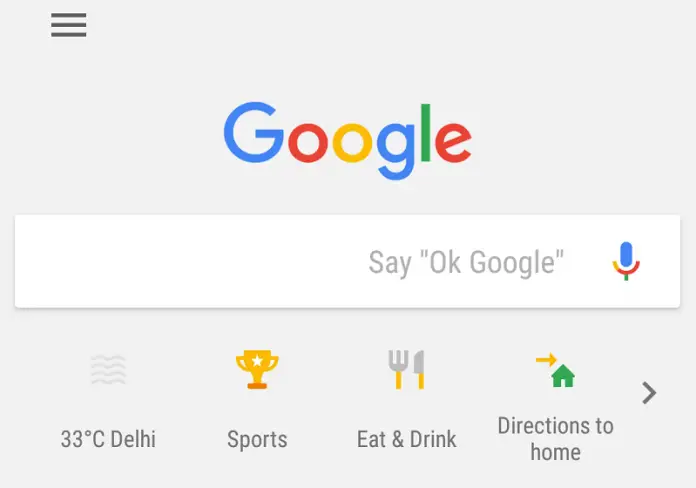The screenshot displays a unique interface of the Google homepage, differing significantly from the traditional versions seen on smartphones and laptops. The central focus is the prominent Google logo, which showcases the familiar multi-colored scheme: a blue "G," followed by red, orange, blue, and green letters. 

Below the logo is a white search bar that includes the phrase "Say 'OK Google'" to prompt voice commands. Adjacent to this prompt is a blue microphone icon. Underneath, the screen displays the current temperature—33 degrees Celsius—in Delhi, accompanied by a weather-related graphic depicting curved lines.

Above this information, a horizontal menu features several categories: a sports section highlighted by a yellow trophy icon, a dining section marked by a fork and knife, and a navigation option symbolized by a green house and an arrow indicating directions to home. To the right of these icons, there is a right-facing arrow suggesting the possibility to scroll for additional options.

In the top left corner, a three-bar icon—also known as a hamburger menu—indicates access to settings or additional features. The overall background of the page is a light gray, giving it a clean and uncluttered appearance. This distinct layout does not fully extend to the top and bottom edges of the screen, making it appear more compressed compared to standard web interfaces.